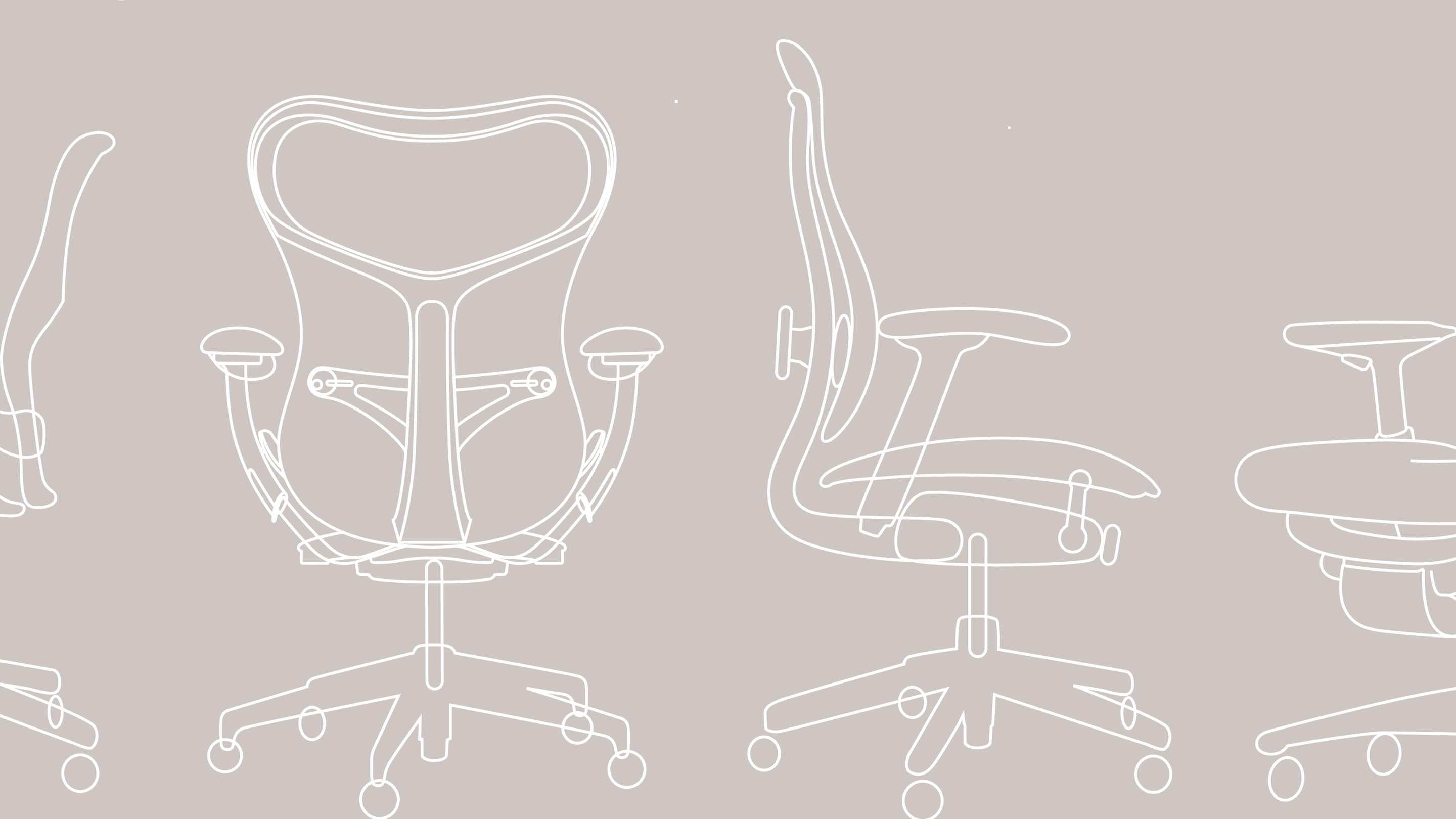This image is a simple, computer-designed drawing of an ergonomic office chair displayed on a background that appears to be a light purple or desaturated red. The image is set within a horizontal rectangle and consists of four distinct outlines of the chair, shown from different perspectives. 

On the far left, the outline depicts the chair facing to the left, partially cut off so that only the rear and caster wheels are visible. Moving right, the second drawing shows a view from behind the chair, where the details of the armrests, back support, and wheelbase are evident. The third outline displays the chair from the right side, highlighting the lumbar support, armrests, cushion, and caster wheels. The final image on the far right is partially cut off, providing a view of the chair from the front with only the right armrest, front cushion, and two caster wheels visible. 

Overall, the diagram uses basic white outlines to illustrate the shape and essential features of the office chair, emphasizing its ergonomic design but lacking intricate details.